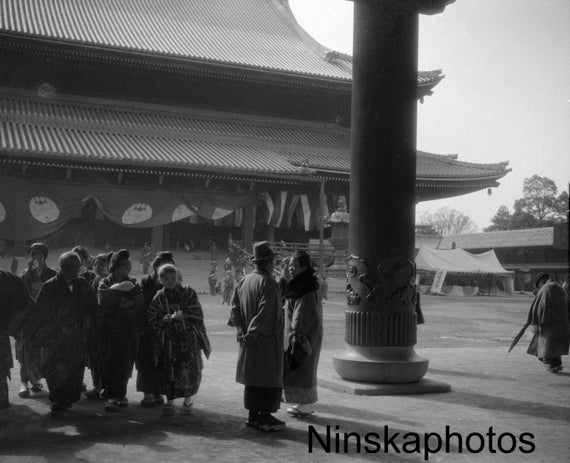This antique black-and-white photograph captures a bustling scene in the courtyard outside a grand Chinese pagoda. The pagoda is an imposing structure with two elegantly tiled roofs that curve upward at the edges. Adorning the lower level of the roof are an array of flags and banners, adding a festive atmosphere to the setting. Numerous people, both sitting and standing, populate the stairways that lead to the pagoda's multiple entrances, suggesting a social or ceremonial gathering.

In the foreground of the photograph stands a giant ornamental pillar, richly decorated at its base. To the left of this pillar, a group of individuals is depicted wearing winter clothes, including thick coats with fur stoles. The women in the group are notably wearing traditional shoes with platform soles, indicative of bound feet. On the lower right-hand corner of the image, the text "Ninska Photos" appears in black font, attributing the photograph to its creator. The composition intricately merges the architectural beauty of the pagoda with the cultural and social elements of the period, offering a vivid snapshot of historical life.